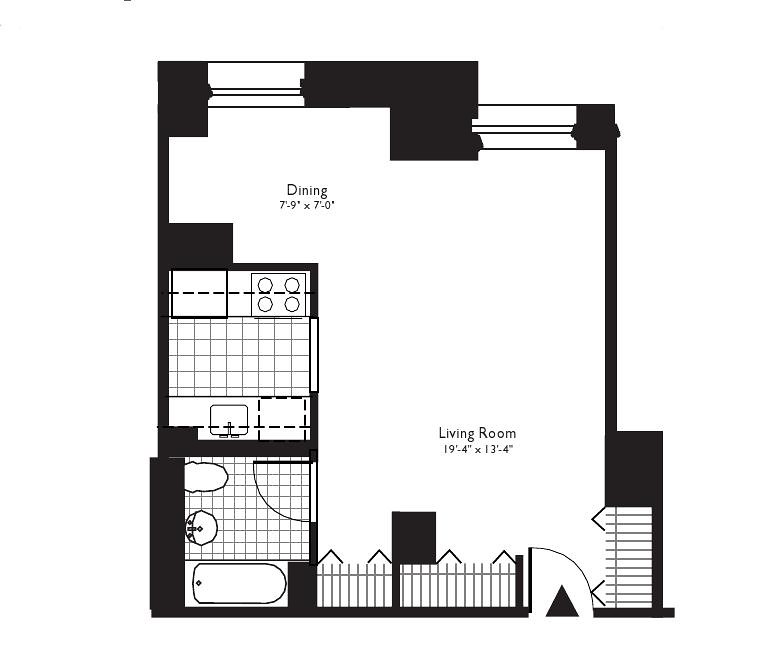The image depicts a detailed blueprint of a rectangular building layout. At the top, there are two designated window spaces. Adjacent to these windows is a marked dining area measuring 7 feet 9 inches by 7 feet. The layout then divides into two distinct sections: the left side features what appear to be the kitchen and bathroom areas, although their specific dimensions are not provided. The bathroom is seemingly a full bath, equipped with a bathtub, sink, and toilet. The right side of the plan, occupying approximately two-thirds of the space, is dedicated to the living room, measuring 19 feet 4 inches by 13 feet 4 inches. The main entryway leads into the living room, and there is an indicated grating or porch area surrounding this entrance.